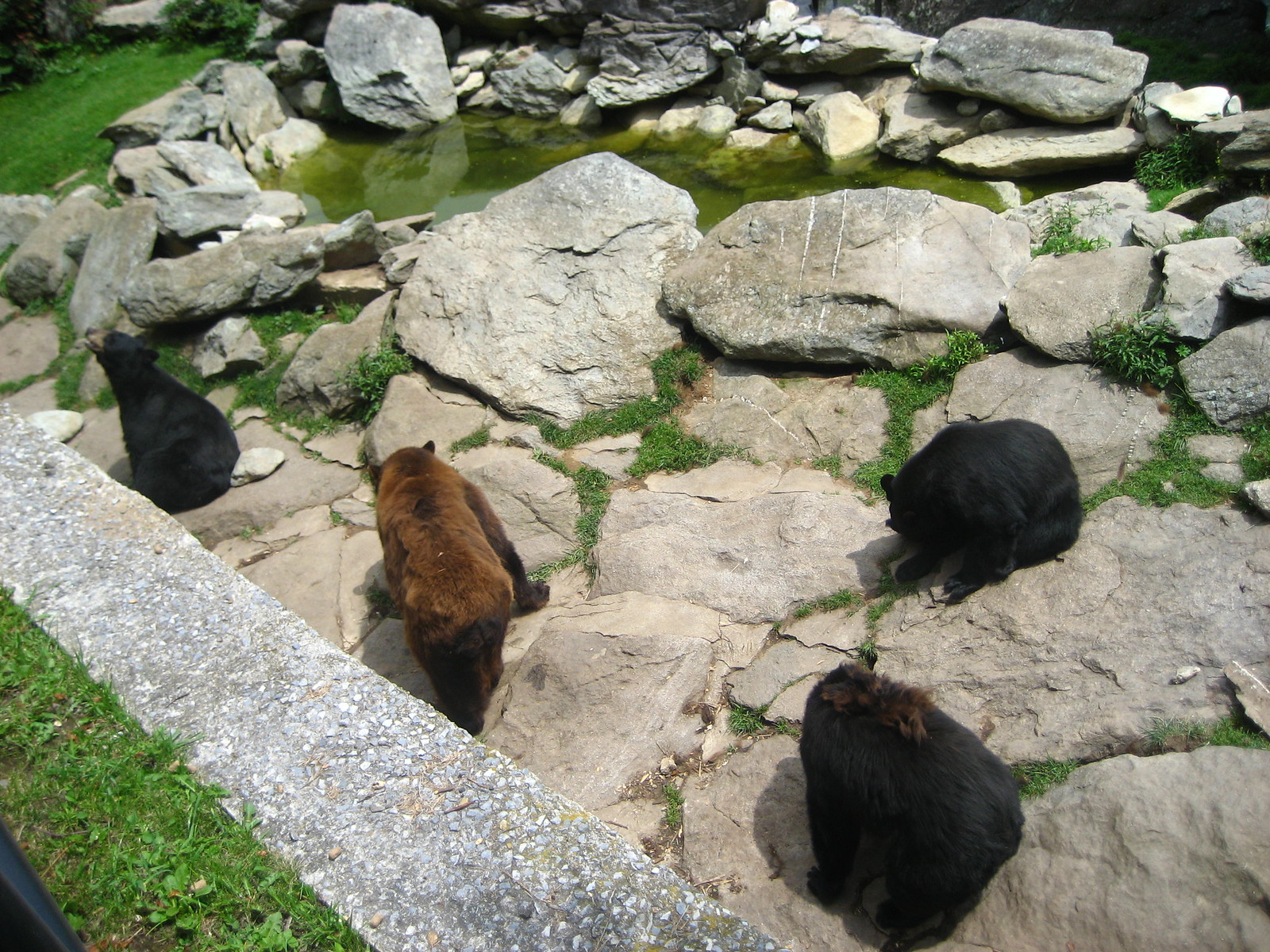The image portrays a rocky, zoo-like exhibit viewed from above, featuring four bears amidst a landscape of gray and beige rocks interspersed with patches of green grass. Three of the bears, positioned to the left and right, are dark brown or black, while the central bear is a lighter brown. The bears appear unusually small, possibly indicating they are young cubs, as they are diminutive compared to some of the surrounding rocks. The rocky terrain is complemented by a murky, green-tinged body of water nestled centrally among the rocks. The viewpoint appears to be from someone standing outside the exhibit, looking down at the bears on a rocky surface. Notably, the image may be AI-generated, as the bears lack realistic details, with one even appearing headless.